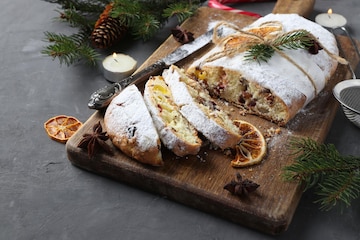This color photograph showcases a beautifully arranged display on a rectangular wooden cutting board with a handle extending out of the frame in the upper right-hand corner. The focal point is an oval loaf of bread or cake, partially sliced into at least three pieces, revealing a yellow interior studded with a variety of nuts, such as pecans, and possibly reddish berries. The confection is generously dusted with white powdered sugar, adding a festive look. A rustic touch is provided by a sprig of pine branch tied on with brown string resting atop the loaf. Scattered around the cutting board are slices of blood oranges and sprigs of green leaves. Additional decorative elements include pine cones and an illuminated white candle in a small cup-like container positioned in the upper right-hand corner of the scene. The backdrop for this arrangement is a gray stone surface, completing the cozy and inviting display.